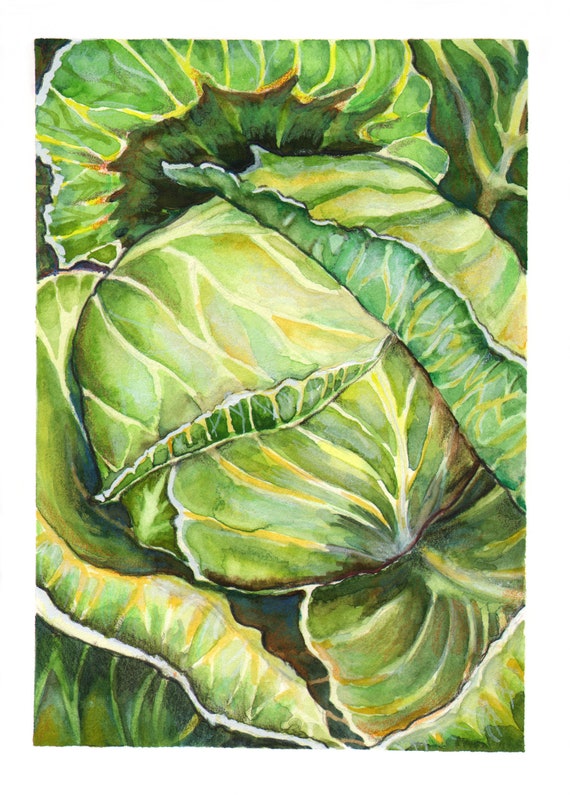This image is a detailed watercolor illustration of a leafy vegetable, likely lettuce or cabbage. The central focus is a full head with surrounding loosened leaves, vividly depicted with layers of rich greens, yellows, and whites, accented by purpling-black shadows near the edges. The veins are intricately painted using white, gold, and yellow, enhancing the texture and depth of the leaves. The illustration captures the nuances of the vegetable with detailed veining and ridges, though the use of broad watercolor strokes adds an expressive and artistic touch. The composition is in portrait mode, offering a close-up view that highlights the natural patterns and color variations within the vegetable's leaves.